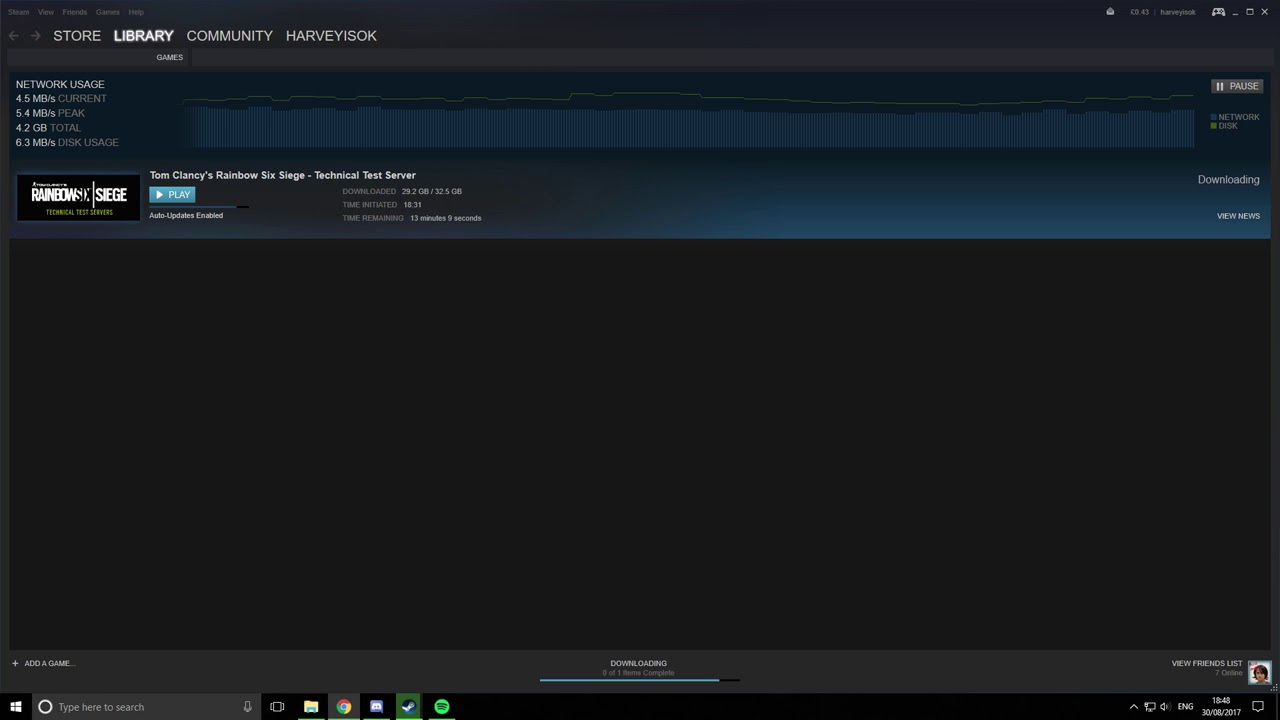This detailed image showcases a computer screen running the Steam client on a Windows operating system. Prominently displayed at the top of the screen are bold, white, capitalized tabs reading 'STORE,' 'LIBRARY' (highlighted), 'COMMUNITY,' 'HARVEY ISOC,' 'GAMES.' Directly beneath these tabs is a detailed panel displaying network usage statistics: '4.5MB current,' '5.4MB peak,' '4.2GB total,' and '6.3MB disk usage,' along with a graph visualizing the bandwidth usage over time. The focal point of the screen is the download progress for "Tom Clancy's Rainbow Six Siege Technical Test Server," with notable details such as a small blue play button and a download progress bar indicating that the download is approximately 80-90% complete. The background remains predominantly black, accented by a dynamic wavelength line. At the very bottom of the screen, the Windows taskbar is visible, displaying an assortment of icons, including Google Chrome and Spotify, alongside the system clock and date.